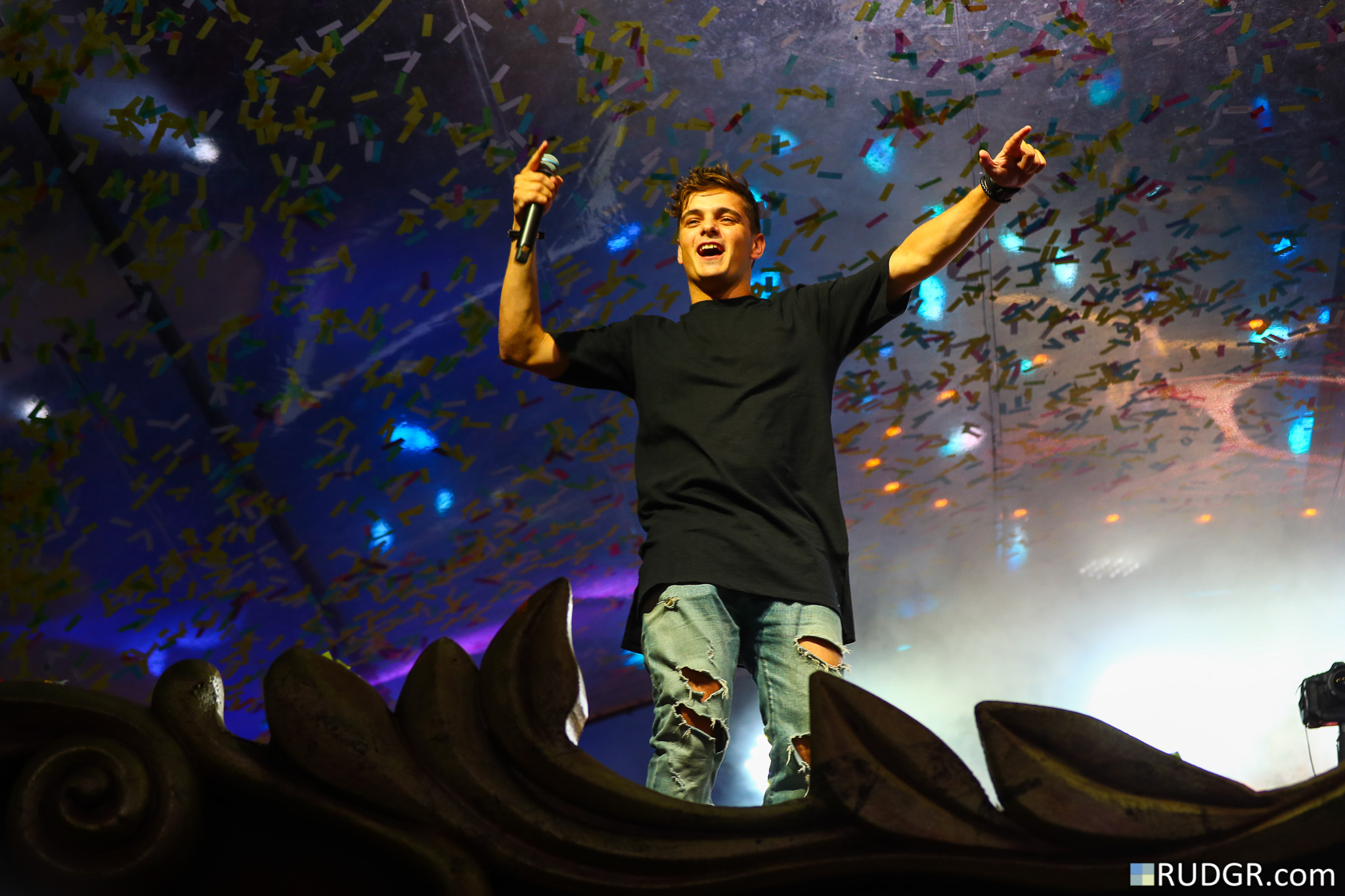A young male performer, likely a lead singer, is captured in mid-performance on stage in this vibrant color photograph, possibly taken by an audience member at a concert event. The singer, who is of white ethnicity with a generous shock of brownish-auburn hair, is seen holding a microphone in his right hand while his left arm extends outward, pointing forward with his thumb and forefinger. He is dressed in a long black short-sleeved t-shirt that extends below his waist, paired with light distressed blue jeans with numerous holes.

The stage features a unique decorative edging at the front, intricately carved into shapes that swing out and upward, resembling feathers. A cascade of confetti falls from the ceiling, adding to the dynamic stage presence. Behind him, an array of colorful lights shines in hues of blue, white, and purple, complementing the large screen displaying visual effects including aqua blue blotches, images of birds in flight, and splotches of orange and dark blue.

The bottom right-hand corner of the photograph features a small, eighth-inch square logo with blue and white colors and the text "RUDGR.COM" in all capital letters, indicating the likely source of the photo. This vividly detailed scene portrays the energy and ambiance of a live musical performance with striking visual elements.